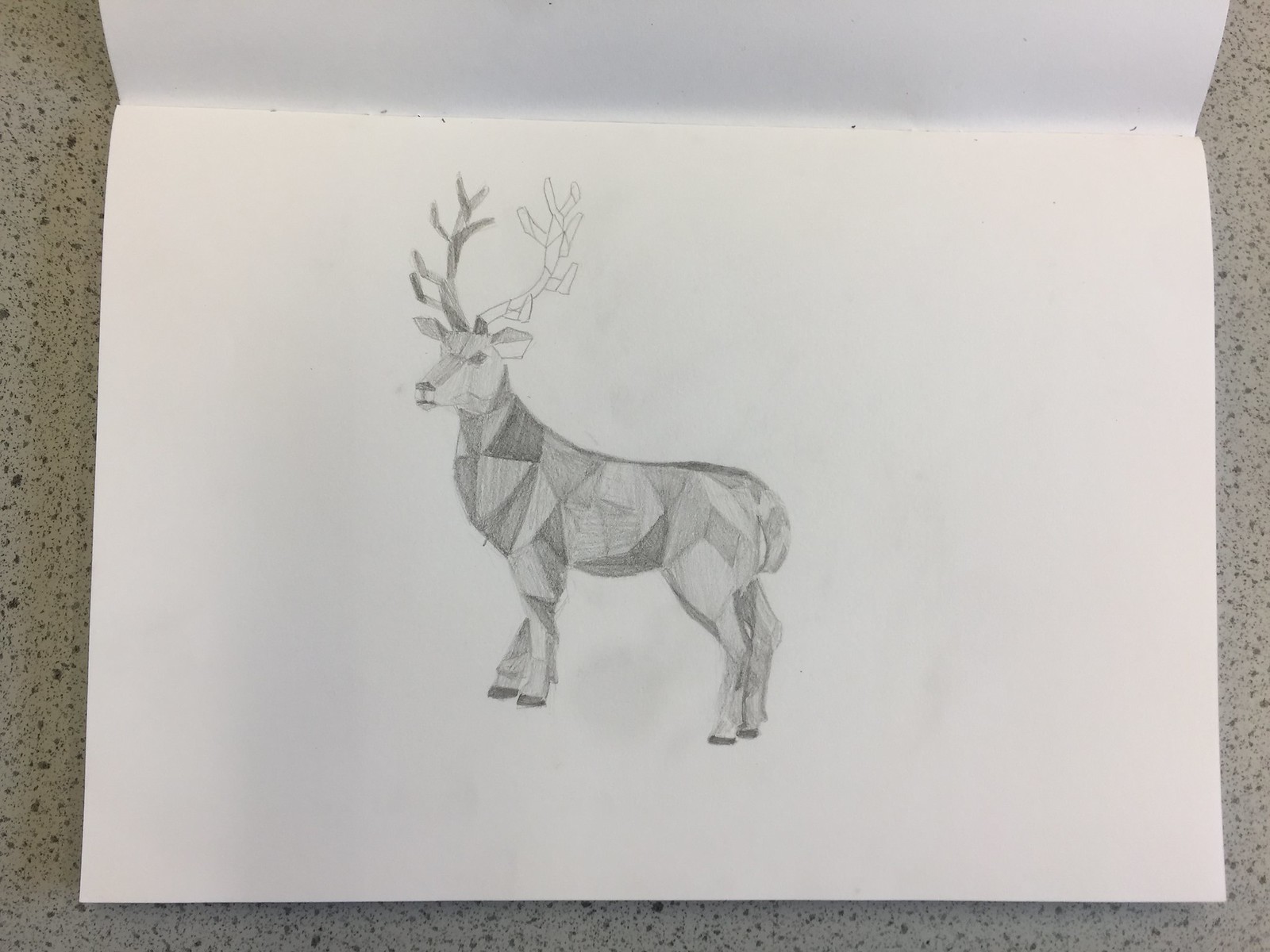This image features a meticulously detailed sketch of a deer, captured from a side angle. The drawing rests on a gray countertop or table, which serves as the background, visible around the entire perimeter of the image. Nestled centrally on this surface is a piece of paper in shades of white and light gray, upon which the deer sketch emerges with remarkable intricacy.

The deer is depicted in profile, showcasing both its front and hind legs. The shading varies in different shades of gray, predominantly light tones, which bring depth and realism to the sketch. On the right side of the deer, its tail is clearly visible, while its face, turned to the left, displays an impressive level of detail. The antlers are particularly striking; the left antler is rendered in a mix of gray and dark gray hues, contrasting with the right antler, which is illustrated in white. The artist's skillful use of shading and attention to detail make this sketch a captivating focal point of the image.